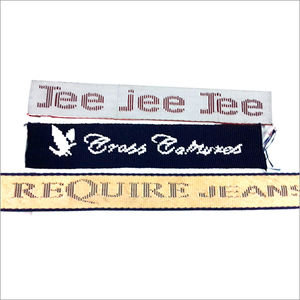The image shows three neatly stacked, fabric banners set against a white background with a thin black lined border. The topmost banner is white with a reddish text, displaying "GGGJEJEJE" in a techy font reminiscent of the 80s, with fine lines running through each letter. The second banner is a dark navy blue featuring a dragon logo on the left and white text that reads "Cross Creatures." The third banner at the bottom has a blue border and a pinkish-cream base color, with the phrase "Require Jeans" in a blue, techy font, similar in style to the top banner. The banners' textures suggest they are made of fabric, given their slight waviness and tactile appearance, making them likely labels or advertisements in a clothing store setting.